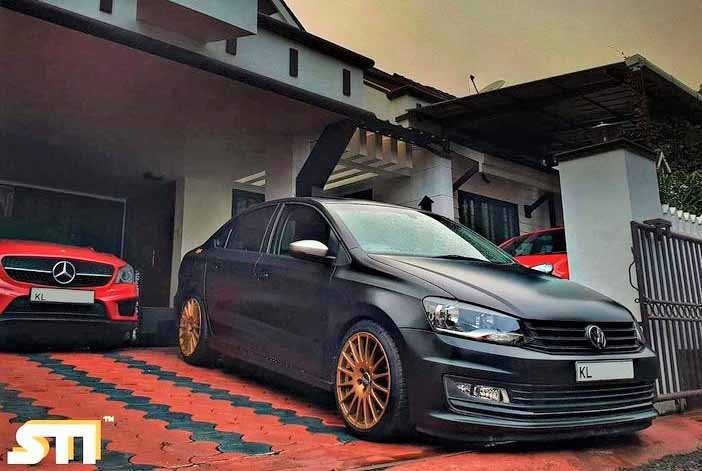This low-angle, landscape-oriented photograph captures the driveway of a white house with white columns under a white awning roof, featuring black edging and detailed vertical slots around its circumference. The image quality is very poor, with noticeable pixelation and discoloration. The driveway, which is inclined at several degrees, is vibrantly colored, predominantly red with black, uneven, swirly lines that run vertically from the back to the front. 

On the right side of the driveway, pointing towards the curb, a dark grey Volkswagen with golden bronze rims is parked, its white license plate displaying black text beginning with "KL". Partially visible behind it is another red vehicle, hinting at another car parked further up the driveway. Additionally, further back to the left under the awning, the front of a red Mercedes with a similar "KL" license plate can be seen. 

Off to the right, a sliding gate is visible but cannot be closed due to the VW's bumper hanging off the driveway. The overall scene is set against the backdrop of a Floridian, Miami-style house, evoking a slightly dusty and sunlit atmosphere.